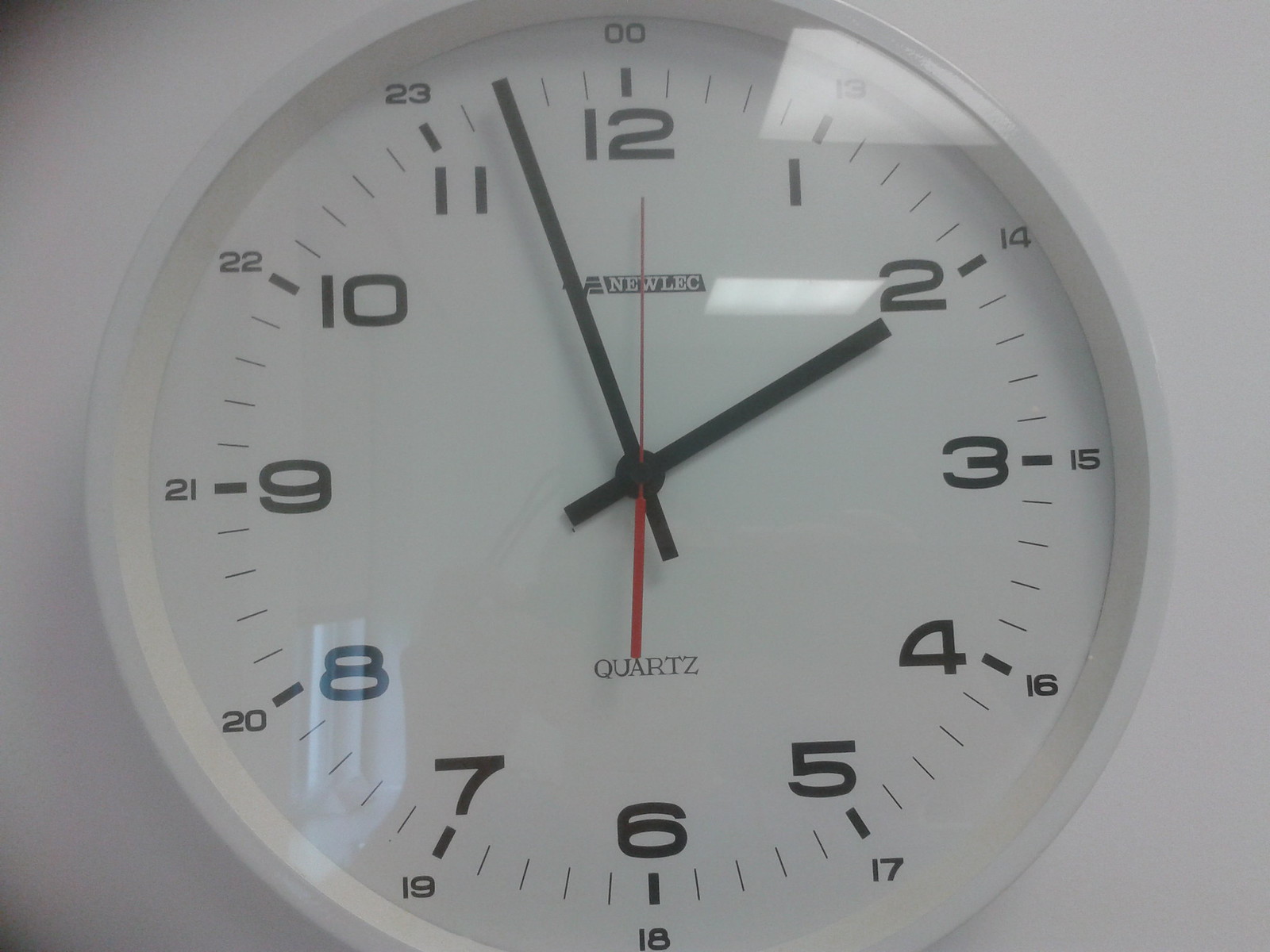This image features a large, white, circular clock, prominently centered against a white background. The clock face is covered with glass, revealing black, modern-font numbers for both the standard 1 to 12-hour markings and an outer ring displaying 13 to 24-hour military time. The clock hands are black, with the shorter hand pointing at 2 and the longer hand positioned between 11 and 12, indicating approximately 1:57. The thin red second hand is precisely on the 12. In the center of the clock, there is a black rectangle with the brand name "Neweck" in white letters. Just above the 6 o'clock position, below the red second hand, the word "quartz" is also printed in black. The clock spans most of the image, extending from top to bottom with about an inch of margin on either side, and there's a notable light reflection at the top of the glass surface.